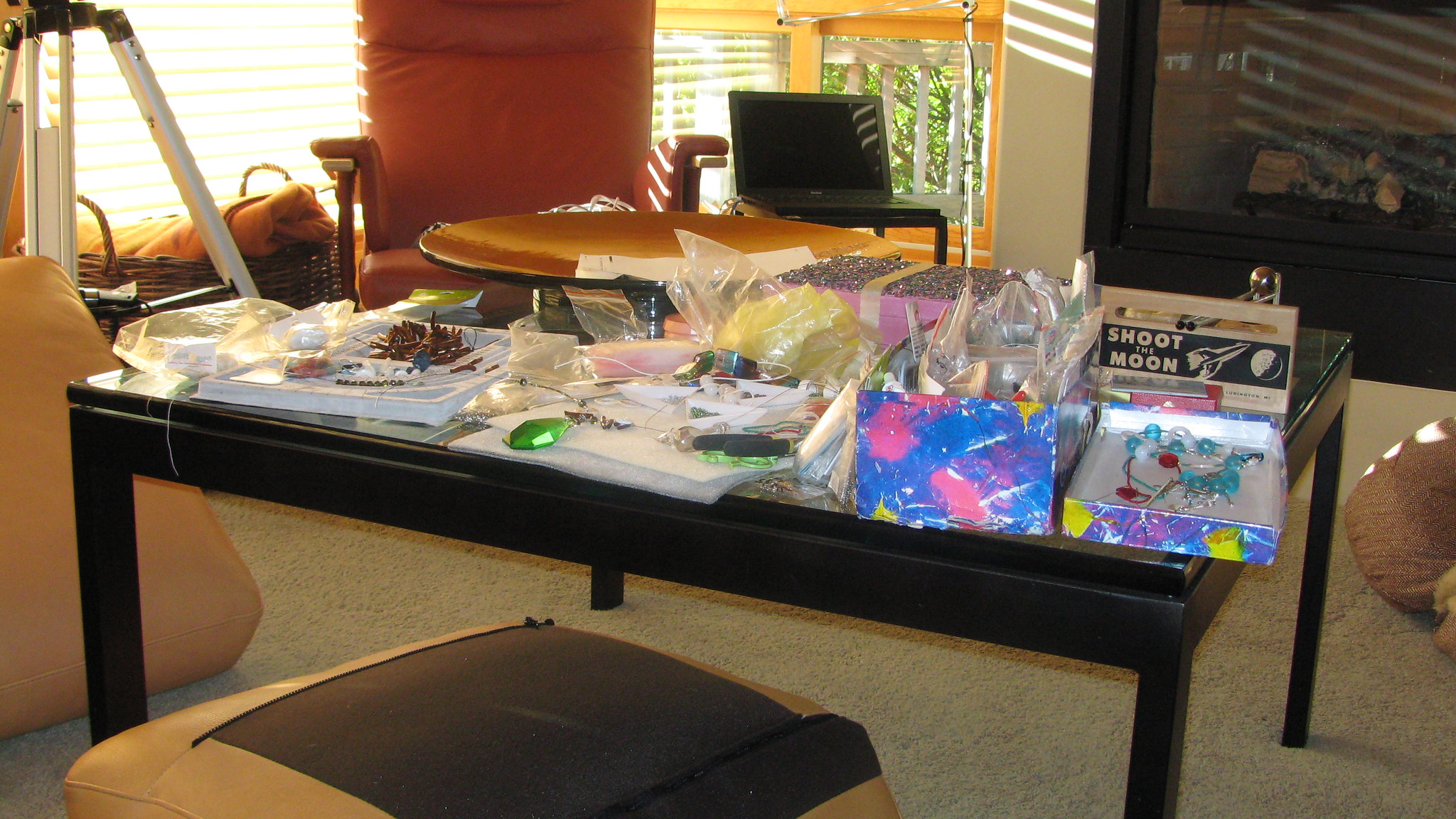In this first-person POV image of a lounge room, the dominant feature is a partially visible black leg rest with brown borders in the foreground. Adjacent to the leg rest is a glass-topped coffee table with steel black lugs, though the glass surface is barely discernible beneath an array of assorted items. Scattered across the tabletop are various papers, craft materials, clear plastic wrappers, and a significant chrome golden bowl-shaped dish positioned at the far left. On the bottom right of the table rests a colorful cardboard box wrapped in purple, pink, and yellow splotted paper, beside which is a stapled cardboard package adorned with the text "shoot the moon" and an illustration of a rocket aiming at the moon.

The coffee table sits on a light brown, white-discolored carpet. In the background, a black-framed fireplace with fragmented wood appears dormant. To the side of the fireplace, a small table—possibly a chair-side or bedside table—supports an open laptop displaying a blank screen. Finally, a brown leather rocking chair is partially visible in the top left corner of the composition, adding to the eclectic and lived-in ambiance of the lounge room.